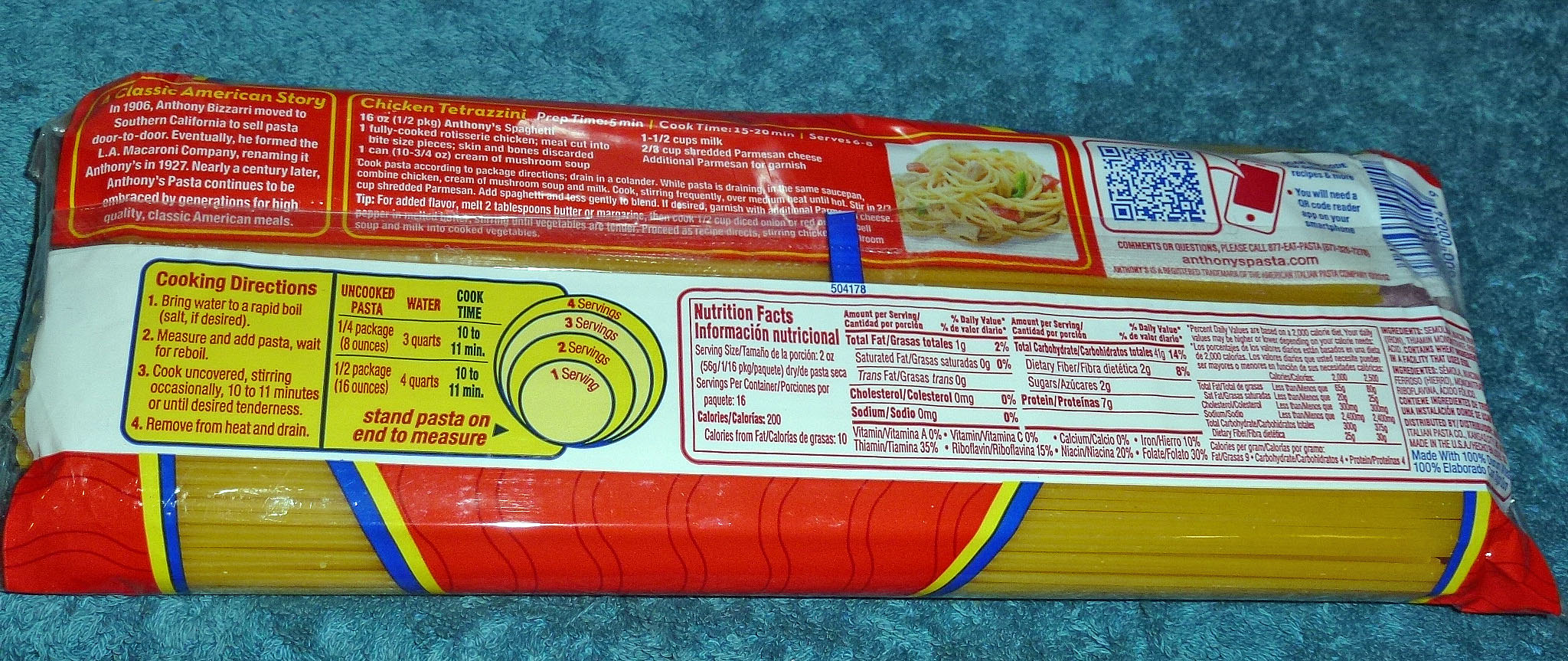This photograph showcases the back side of a spaghetti pasta package. The packaging features essential information such as cooking directions, nutritional facts, and suggested recipes for preparing the pasta. The package is displayed against a textured blue surface that appears to be made of a soft, fabric-like material, possibly felt, satin, or silk, rather than a hard surface like wood or stone. The overall layout on the packaging is structured and informative, catering to the needs of anyone planning to prepare a meal with the enclosed spaghetti.